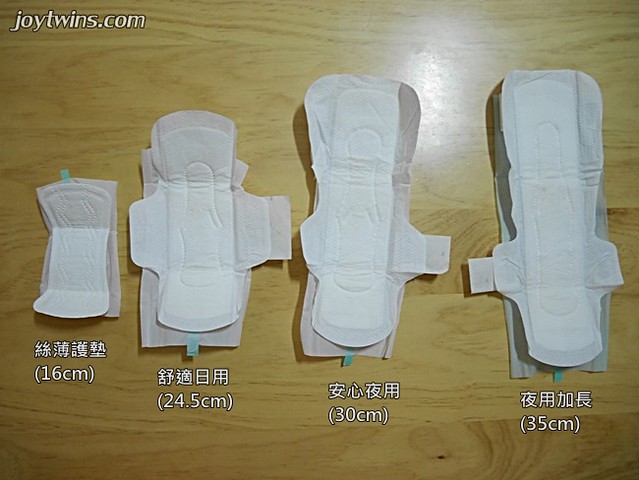This overhead photograph displays four women's pads arranged vertically side by side on a brown table. The top left corner features white text that reads "joytwins.com." Each pad is labeled with its respective length in centimeters and Chinese characters. The smallest pad on the left measures 16 cm and lacks wings. The second pad measures 24.5 cm and includes wings. The third pad is 30 cm long, also with wings, and the largest one measures 35 cm and includes wings as well. All four pads are white with a similar design.